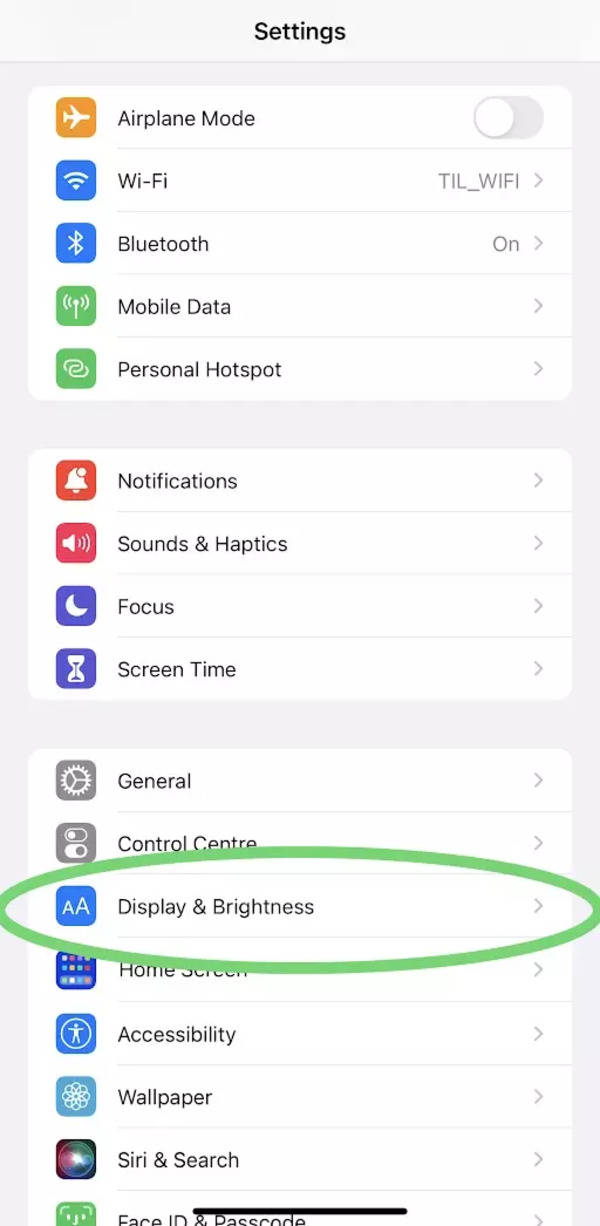This screenshot presents a vertically oriented view of the iPhone's settings menu. At the top, Airplane Mode is displayed with a gold airplane icon in the center, and the toggle switch is set to "off." Below Airplane Mode, there are several options with colored icons indicating their status:

- Wi-Fi: A blue square
- Bluetooth: A blue square
- Mobile Data: A green square
- Personal Hotspot: A green square

Further down, notifications are on, shown by a red alarm icon. The Sounds option features a red square with a microphone icon. Focus is represented by a purple square with a moon icon, and Screen Time has a purple square with an hourglass icon.

Below these options is the General setting, depicted by a gray square with a gear icon. Next, the Control Center is shown with toggle icons. The Display & Brightness option is highlighted by a green circle and marked by a blue square containing two capital A's, with one being smaller.

Following these, the menu includes Home Screen and Accessibility settings, each accompanied by right-pointing arrows indicating they lead to further options.

Each setting is distinctly marked with symbols and colors, providing a clear and detailed overview of the iPhone's configuration capabilities in this particular screen capture.